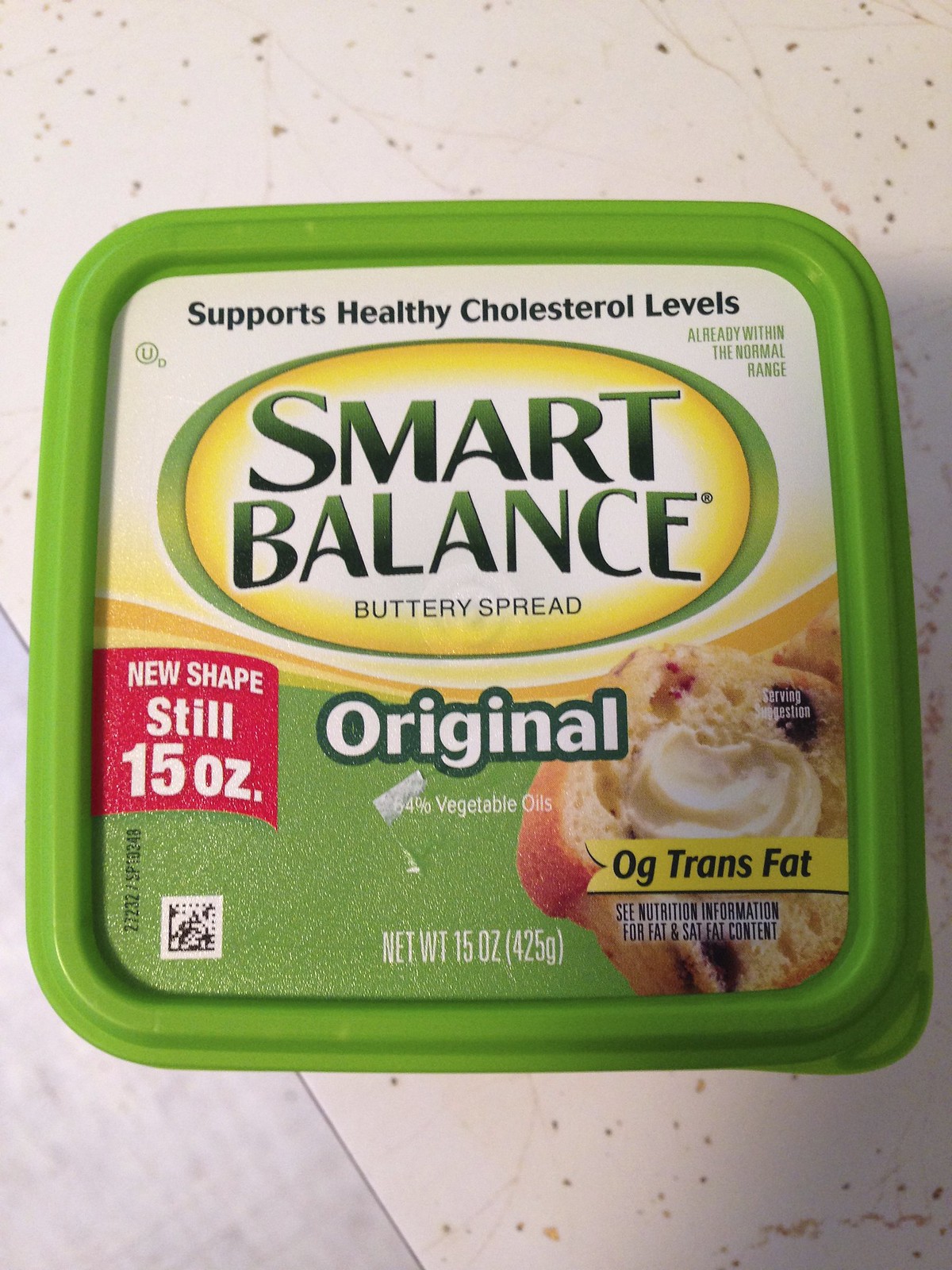In this vertical rectangular image, we observe a surface that may be a table, countertop, or tile floor, featuring a beige background with golden flecks. Prominently positioned on this surface is a square container with a green exterior. The container's lid is adorned with a beige, yellow, and white label. In the center of the label, within a yellow oval, green text reads "Smart Balance Buttery Spread," with "Original" written below it. In the lower right corner of the label, there is an image depicting a slice of raisin bread topped with a dollop of the buttery spread. Above the image, text indicates "0 grams trans fat" and advises checking the nutritional information for fat and saturated fat content. The label also states the net weight of the product, 15 ounces, at the bottom center.